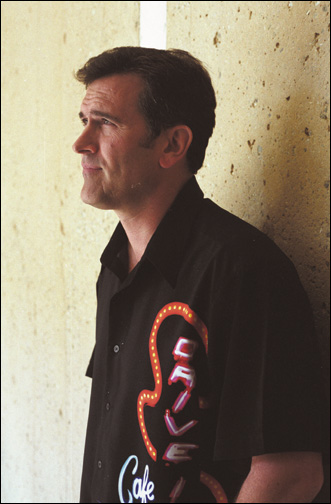The image features Bruce Campbell, captured in a professionally taken, in-focus photograph. He is posing intentionally against a yellow-speckled wall with holes, giving the appearance of being deep in thought. The shot highlights his profile, showing him looking to the left side of the picture. Bruce Campbell appears younger in this image, possibly in his 40s or 50s, with short, dark brown hair and peach skin. He is wearing a black button-down shirt adorned with vibrant designs in various colors – black, white, brown, orange, red, yellow, hot pink, pale bluish white, and tan – that feature the words "drive" and "cafe." The wall behind him is the only background element, emphasizing the deliberate and posed nature of the shot, reminiscent of a promotional photograph.